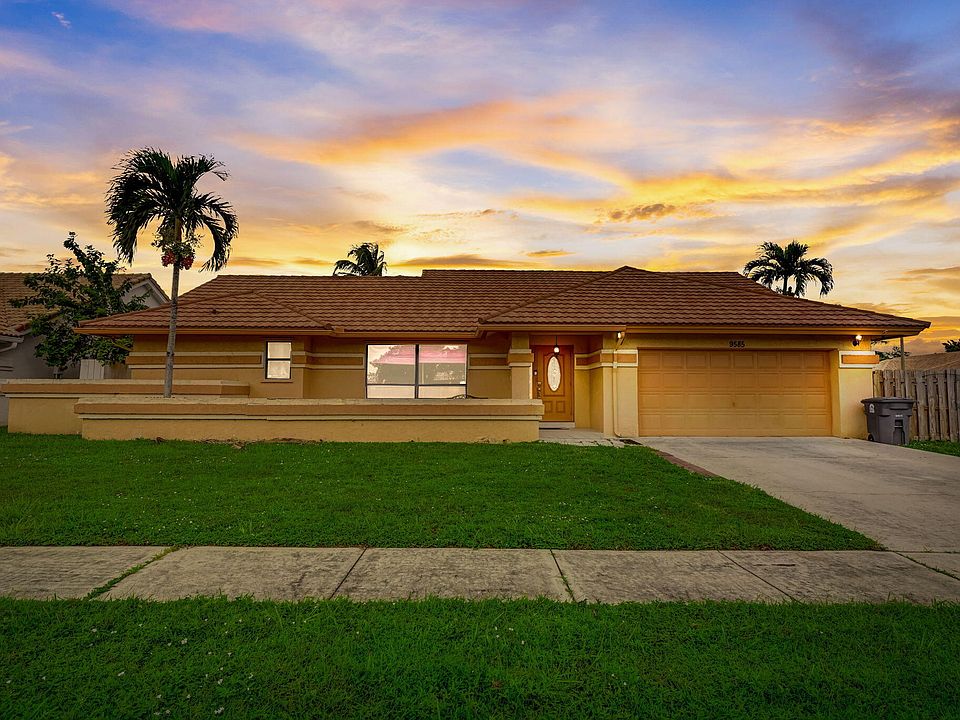This image captures a modern ranch-style, one-story house likely situated in Southern California or Florida, characterized by its recent construction and contemporary details. The house has light tan walls with a contrasting light orange garage door. The lawn in front is well-maintained but could use a trimming. It is adorned with palm trees strategically placed: one to the left of the house, another behind it in the middle, and a third on the right side, suggesting an artificial appeal. 

A single black trash bin is positioned to the right of the garage near a side gate, contributing to the modern and tidy aesthetic of the property. The front door features an oval semi-transparent window, adding a touch of elegance. A small brown fence marks the boundary of the backyard while a shorter brick wall forms a cozy patio area in the front.

The setting sun casts a warm glow on the scene, with yellow and orange hues painting the sparse clouds in the sky, hinting at a serene sunset. The final daylight illuminates the sand-colored walls and the dark orange-brown roof shingles, creating a picturesque ambiance. The driveway and adjoining sidewalk are empty, emphasizing the peaceful, suburban location with enough distance between this house and its neighbors to ensure privacy.

The entire composition, from the manicured lawn and palm trees to the subdued sunset and clear sky, conveys a tranquil and inviting residential atmosphere, making it a desirable place to live.